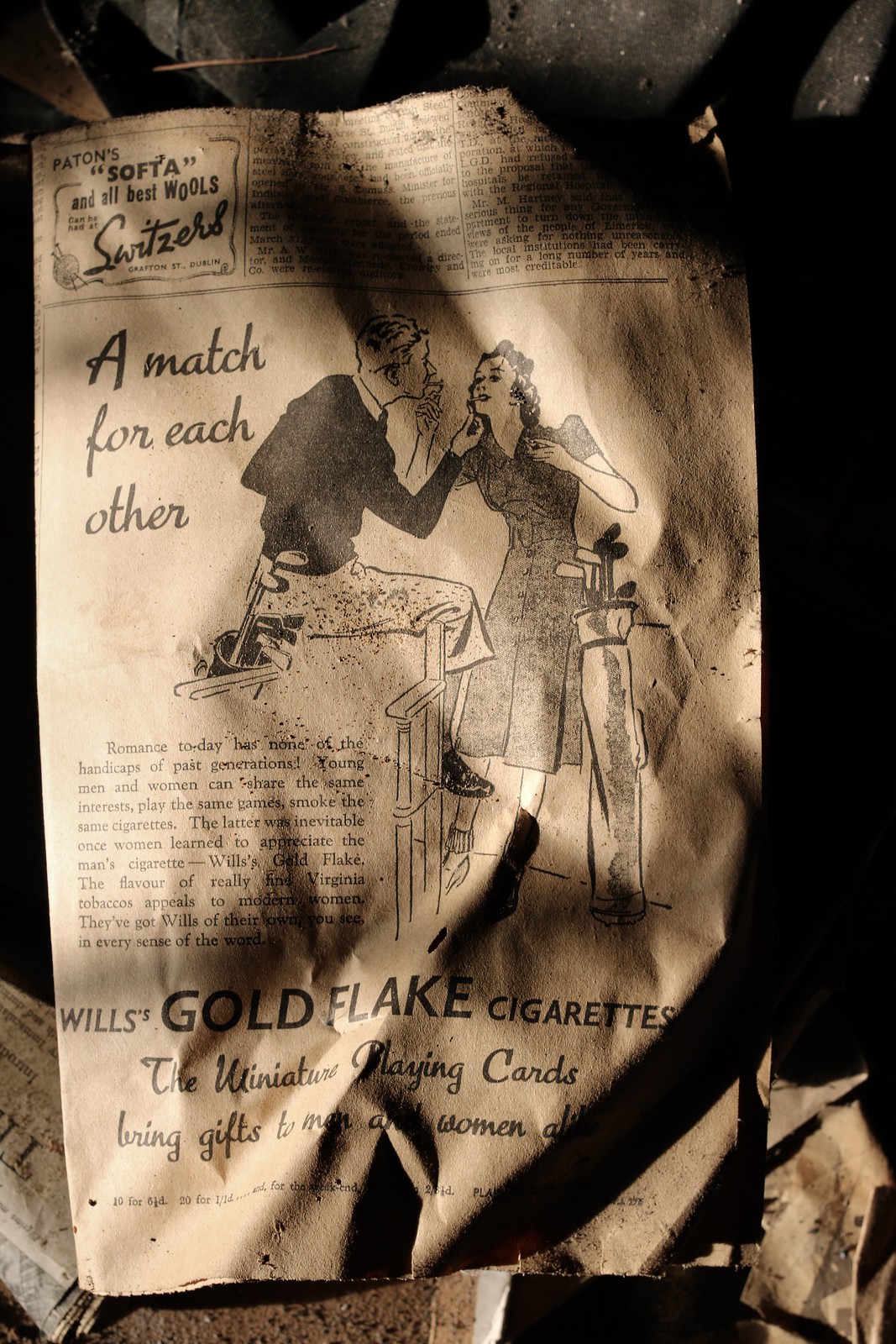The image captures an aged and crinkled piece of newspaper, characterized by its light brown and black tones, possibly due to its age. Dominating the page is a nearly full-page advertisement for Will's Gold Flake Cigarettes. The central artwork features a man and a woman, each lighting a cigarette for the other in an intimate gesture reminiscent of feeding each other cake at a wedding. Both are equipped with golf caddies, with the man sitting on a ledge, gently touching the woman's face as she mirrors his action. Text on the top left reads "Patents 'SOFTA' All Best Wools", while the bold headline to their left states "A Match for Each Other." Further down, it reads "Romance today has none of the handicaps." The corners of the newspaper are heavily worn, creased, and degraded, with visible debris and possible burn marks, adding to its vintage and deteriorated appearance.